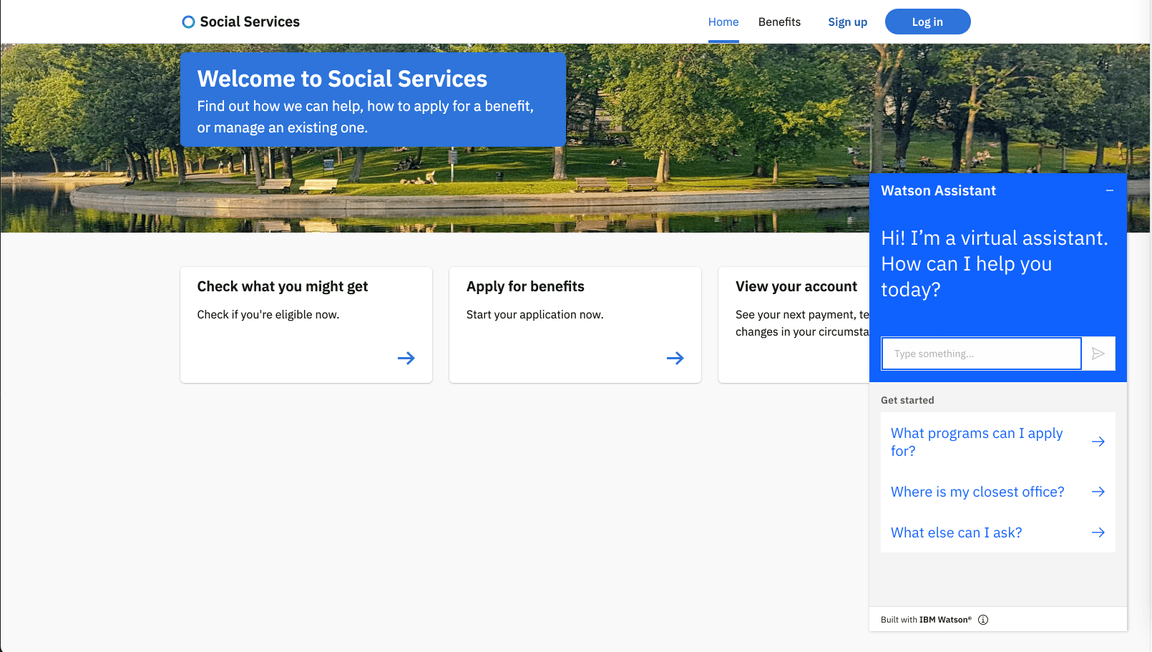The image depicts a subsection of a social services website, likely government-related, aimed at assisting individuals with benefits. The main greeting reads, "Welcome to Social Services," and prompts users to find out how they can get help, apply for benefits, or manage existing ones. On the right side of the screen, a Watson virtual assistant has popped up with a text field, ready to assist users with their queries. The interface includes a set of quick links such as "Get Started," "What programs can I apply for?", "Where's my closest office?", and "Who else can I ask?".

Additionally, the site features several large buttons or links that guide users through various actions: "Check what you might get," "Check if you're eligible," "Apply for benefits," and "View your account." At the top right corner of the page, there are prominent "Sign Up" and "Login" buttons. The user interface predominantly uses white and light gray tones with some blue elements for contrast, creating a clean and organized look.